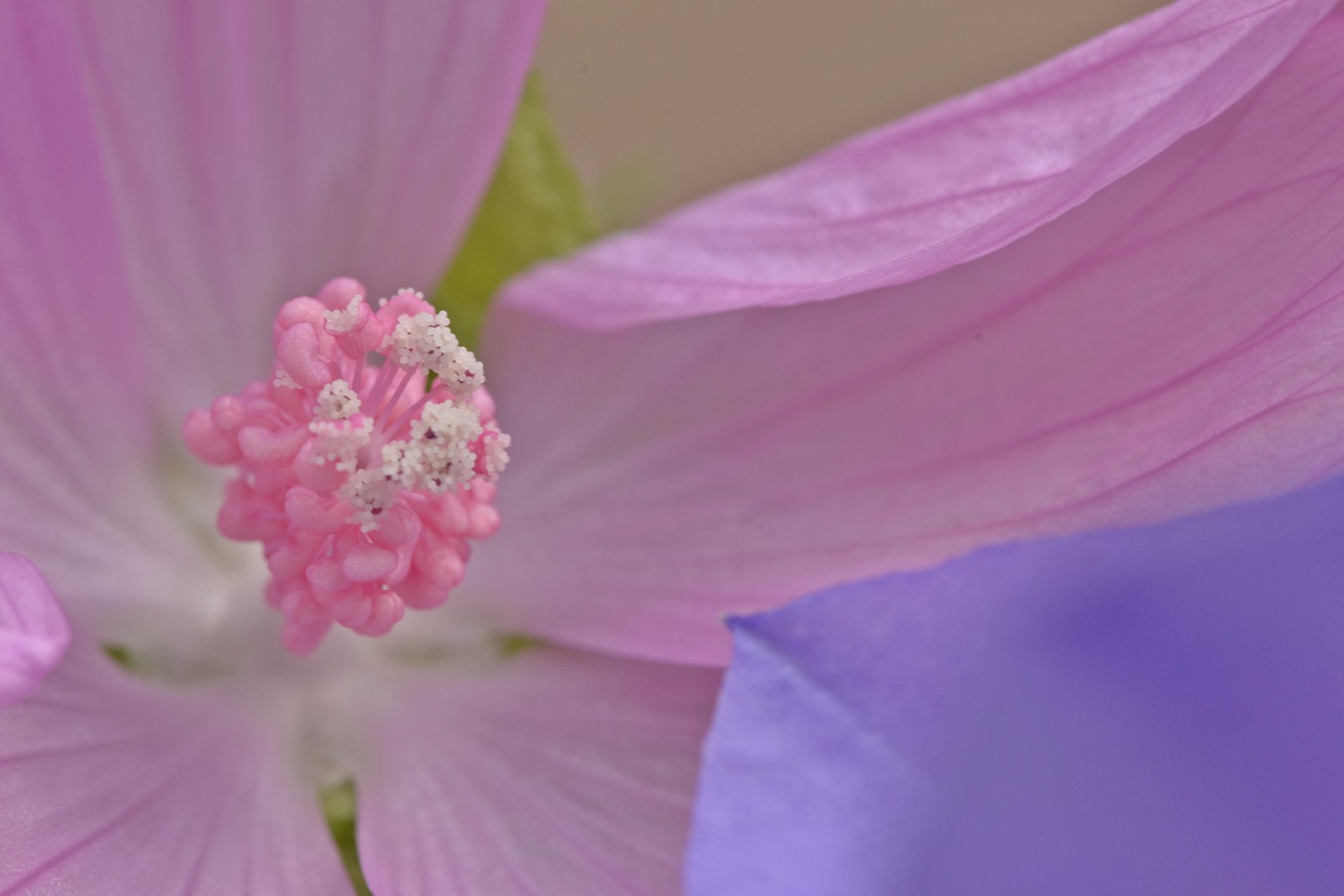This detailed photo showcases a close-up view of a delicate flower, emphasizing its light pink petals which almost appear translucent and feature darker pink veins. The central focus reveals the flower's pistil—a cluster of pink, bean-shaped structures adorned with white specks, likely pollen. One petal in the top right corner is notably folded inward. The image also captures a fragment of another flower in the bottom right corner, distinguished by its more purple hue, suggesting it is a nearby similar bloom. The background is a mix of green, possibly stems or grass, and additional soft purple shades, potentially indicating a second flower or leaves. This setting hints at an outdoor location, possibly a garden or planter near a house or building. The overall pastel palette creates a visually soothing scene, capturing the intricate beauty of these flowers.